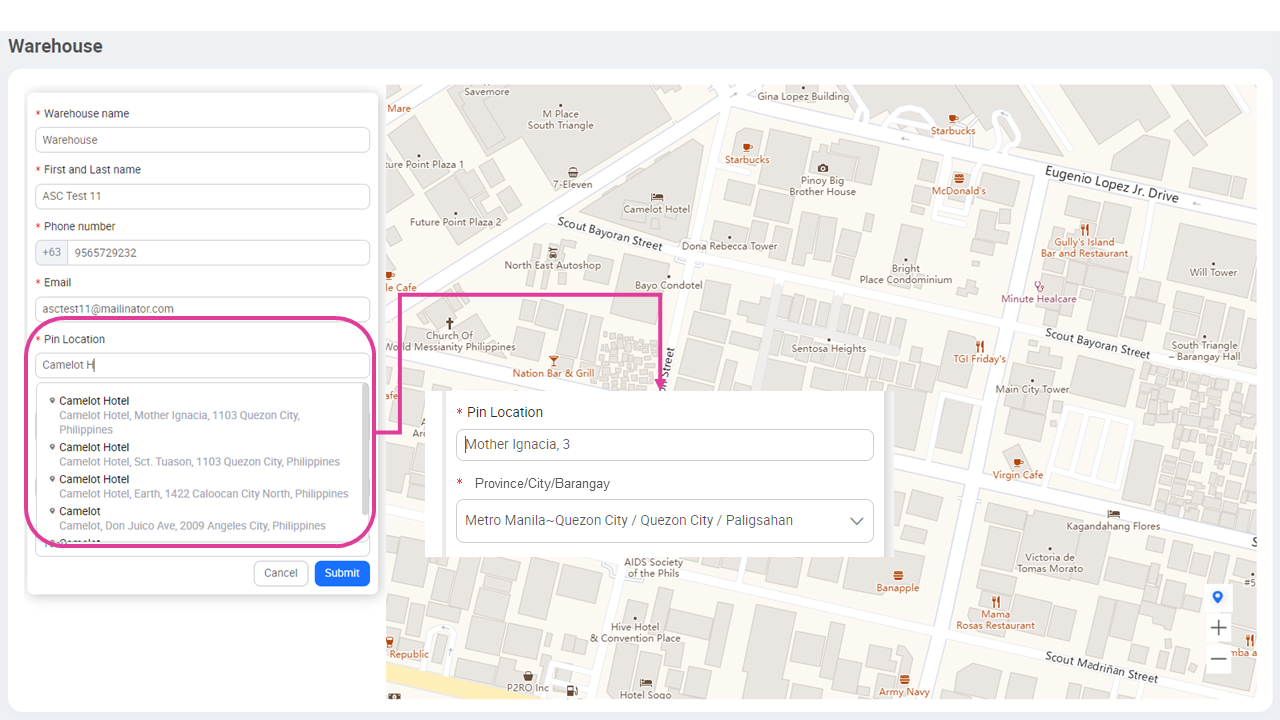In this image, the right-hand side of the page features a detailed map, likely generated through a search query. This map is used to pinpoint locations and is highlighted by a red arrow. On the upper left-hand corner, the bolded text reads "Black Warehouse."

The left-hand side of the image is dedicated to a form interface. In this form, users are prompted to enter several required details, as indicated by red asterisks. The fields in the form include:

- Warehouse Name: "Warehouse"
- First and Last Name: "ASC Test 11"
- Phone Number with Country Code: "+63 9565-729-232"
- Email: "asctest11@malinator.com"

Below these fields, there's a section titled "PIN Location," where the user is typing "Camelot Hotel." This action highlights several possible locations on the map to the right. Each possible location is highlighted in red and linked to the map with an arrow. There is also an additional section labeled "PIN Location in Province City," providing further context for the geographical pinning within the application.

This detailed caption describes the interface elements and user actions captured in the image, providing a clear understanding of what is being depicted.